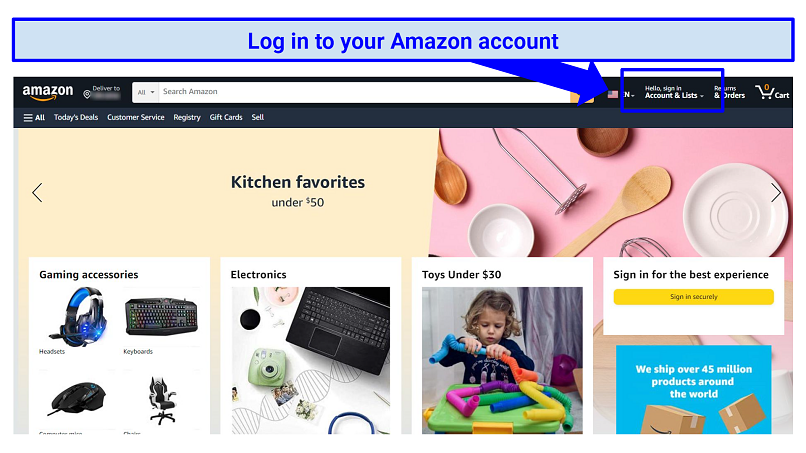The Amazon homepage features a prominent blue banner at the top with a dark blue border that reads, "Log into your Amazon account," highlighted by a blue arrow pointing toward the "Hello, Sign in, Account & Lists" section. This area is encased in another blue box. To the right, you see options for "Returns & Orders," and an orange zero indicating an empty shopping cart. 

On the left, there is a search bar labeled "Search Amazon" with a blurred "Deliver to" section, followed by the Amazon logo. Below this header, there's a navigation bar with links to "Today's Deals," "Customer Service," "Registry," "Gift Cards," and "Sell."

The main content of the front page features various categories:
- "Kitchen favorites under $50" with an image of a spatula and plates.
- "Gaming Accessories," showcasing categories like headsets, keyboards, mice, and chairs.
- "Electronics," with an image of a laptop and a camera.
- "Toys under $30," featuring a young girl assembling colorful tubes.

To the right, a message prompts users to "Sign in for the best experience" with a yellow "Sign in securely" button. A statement below emphasizes that Amazon ships over 45 million products worldwide.